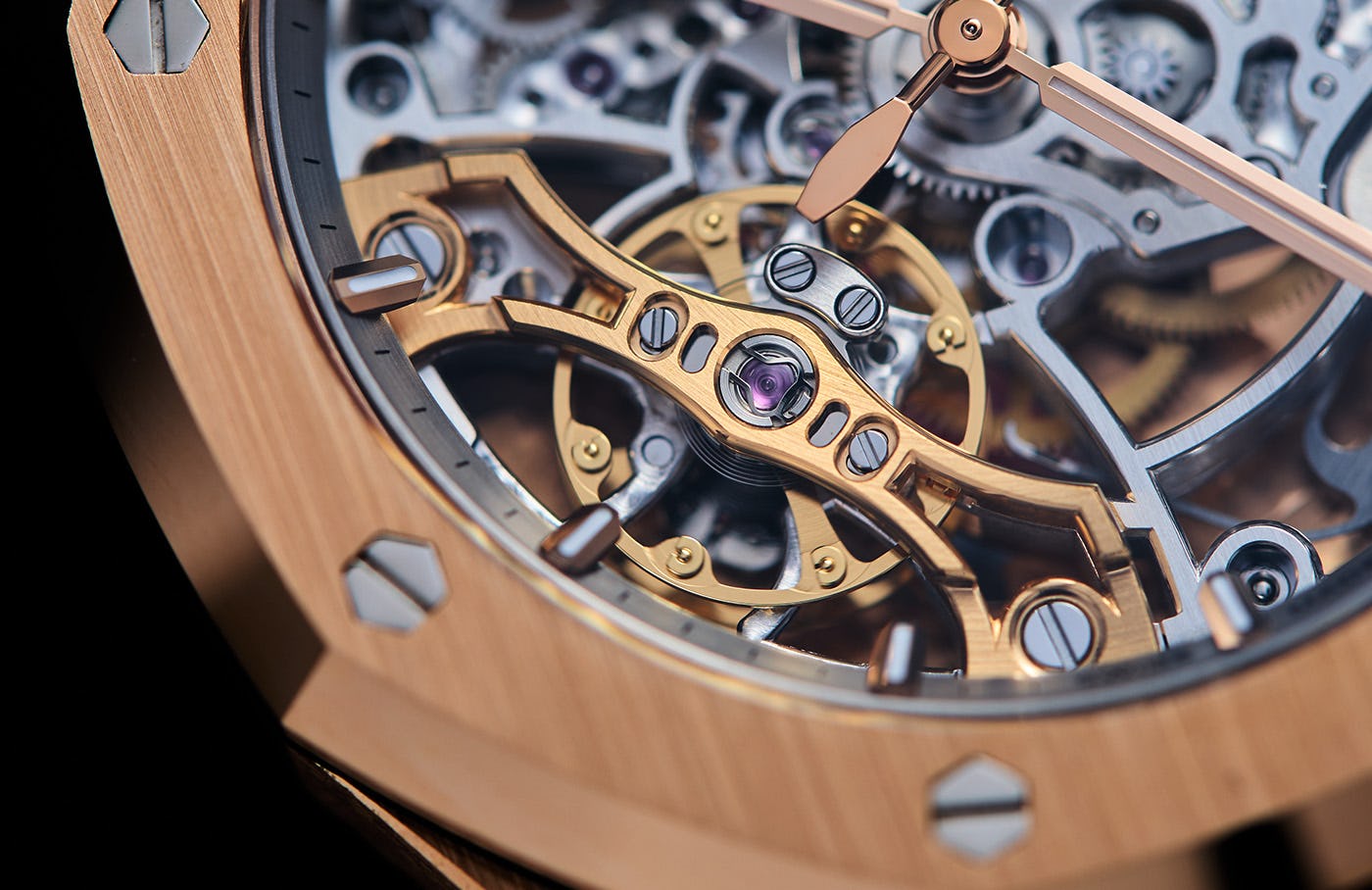This close-up photograph captures the intricate details of a disassembled wristwatch, showcasing its internal mechanics. Dominating the background are a series of interlocking silver and golden gears, highlighting the complexity of the watch's movement. In the bottom left corner, there's a prominently golden, circular metallic part. At the center of this detailed view, there's a purplish jewel, indicative of the watch's jeweled movement, which appears light purple in color, resembling a camera lens. The main hands of the watch, including the hour, minute, and second hands, are visible, with the hour hand being a golden-copper hue. Surrounding the exposed workings, the watch's border features a light wooden finish, complete with hexagonal, countersunk screws. This wooden border displays a fine grain and adds a touch of elegance to the overall mechanical appearance. Dark edges frame parts of the image, hinting at additional wooden components that house the watch. This image perfectly encapsulates the melding of precise engineering and refined aesthetic design.